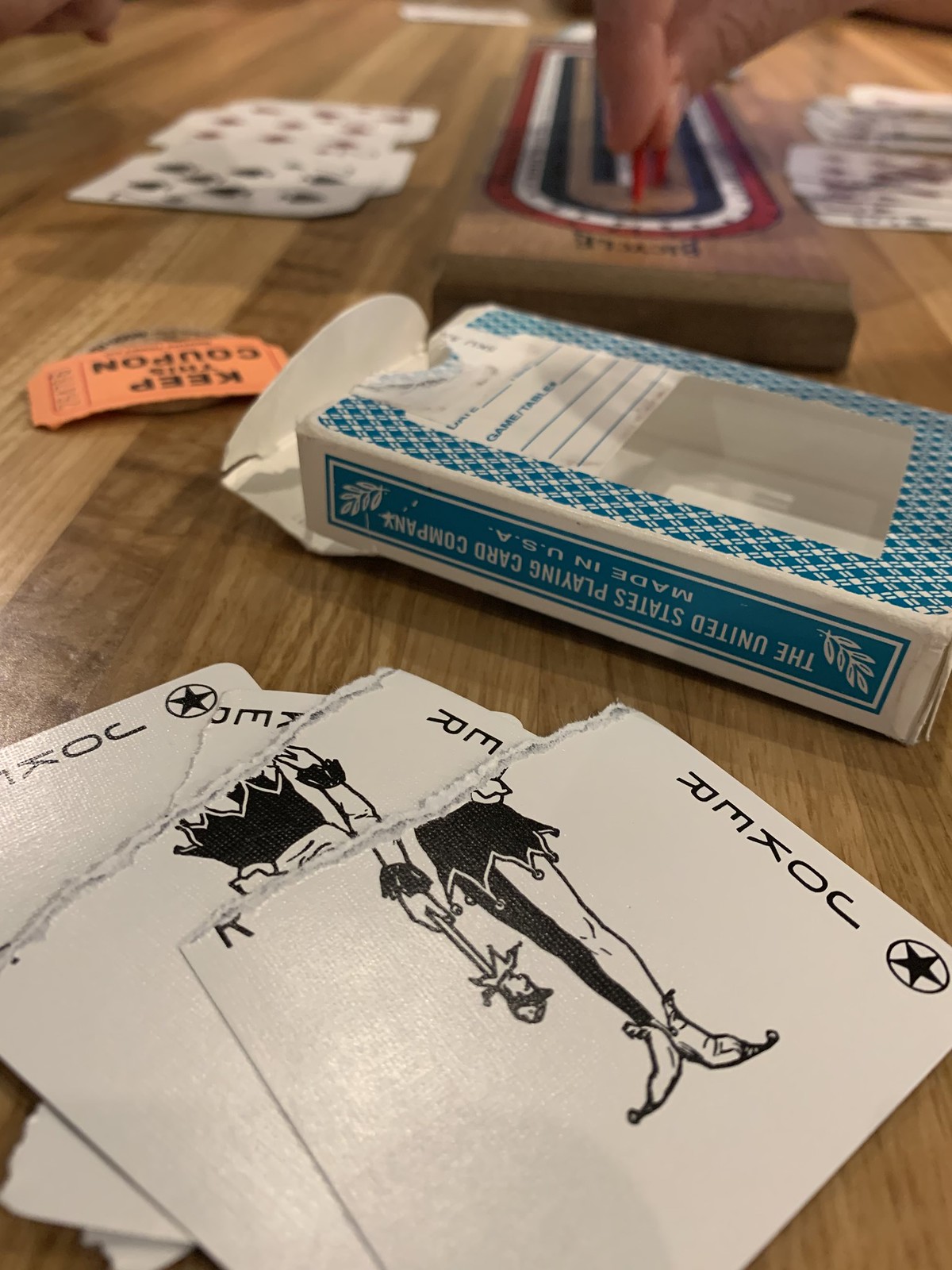This photograph captures an intricate scene of a card game in progress on a wooden table. The table, showcasing a light brown wood grain with vertical slats, fills the entire frame from top to bottom and left to right.

Central to the image are several torn joker cards arranged haphazardly. One prominent joker card, coming from the right side and positioned on top, features a circle and star design in the corner, with the bottom of a jester's clothes visible. Adjacent to it, more partially visible joker cards create a chaotic yet intriguing pattern, with corners and edges peeking out from various angles.

Towards the upper right, a partially open white and light blue card box lays diagonally, revealing a small circle through its opening. Positioned above the card box is a small, orange ticket stub, possibly for a movie theater, bearing the upside-down words "Keep Coupon" in black lettering.

Adjacent to these items, a long, cylindrical piece of wood decorated with spiraling red, white, and blue stripes runs horizontally across the scene. A person's hand, entering from the top right corner of the frame, is seen placing a small red peg into the striped wooden object, with fingers and thumb visible, emphasizing their careful action.

Scattered across this busy tabletop are playing cards, adding to the lively and dynamic atmosphere of the card game in progress.